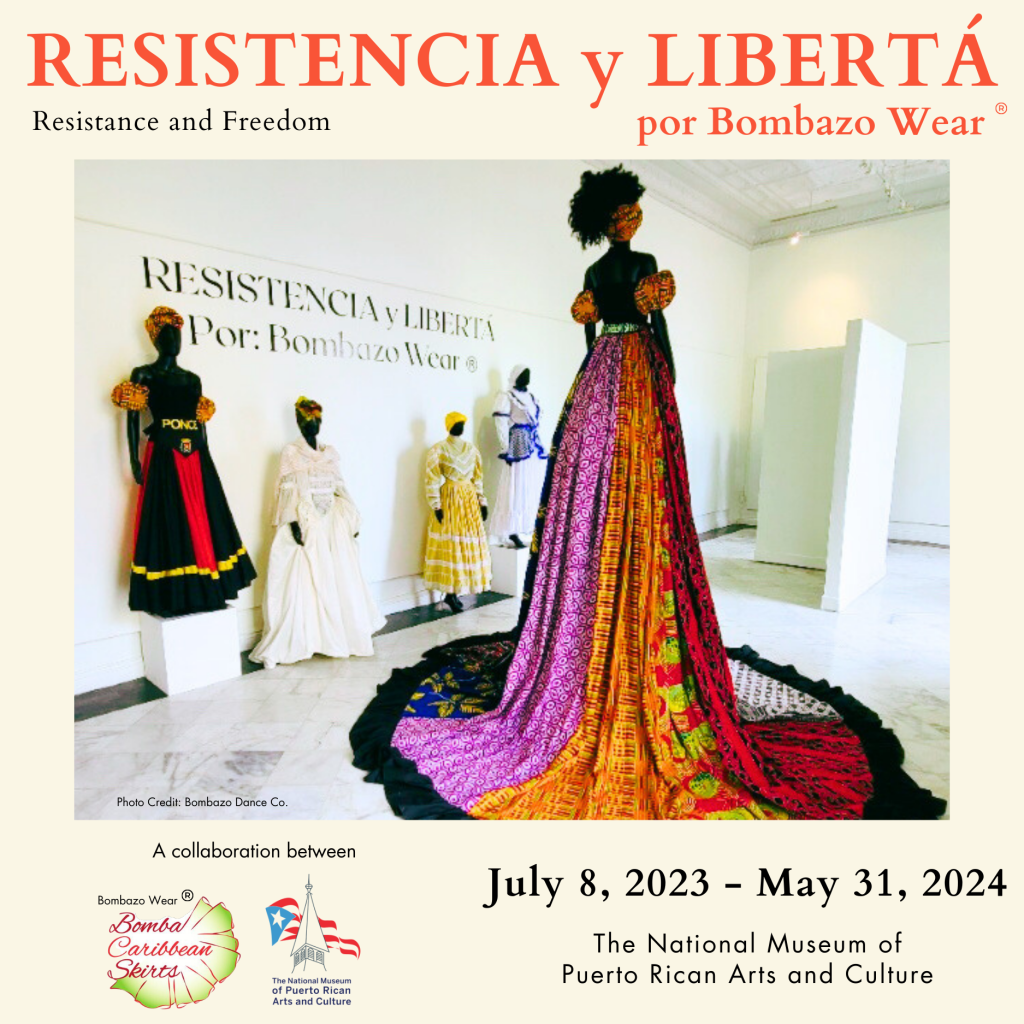The image announces an exhibition titled "Resistencia y Libertad" by Bombazoware, taking place at the National Museum of Puerto Rican Arts and Culture from July 8th, 2023 to May 31st, 2024. The announcement features red block lettering at the top, with the title and its English translation, "Resistance and Freedom," prominently displayed. 

In the photograph, various outfits are showcased on black mannequins. These outfits, seemingly all for female figures, prominently feature long skirts or dresses that reach down to the feet of the mannequins. A striking piece in the foreground is a very tall mannequin, possibly on stilts, dressed in a fantastical, multi-colored skirt made up of fabric strips in shades of pink, orange, red, green, and black lace overlay. The overall appearance of this skirt gives it a dramatic and whimsical flair as it extends approximately 10 feet from the waist to the floor.

The gallery environment is characterized by white walls and directional can lighting from the ceiling, creating a clean and focused display space. The border at the bottom of the image indicates additional information: the photo is credited to Bombazoware Dance Company, hinting that these might be costume pieces for dancers. Text along the bottom also mentions the collaboration between Bombazoware, Bomba Caribbean Skirts, and the Ministry of Puerto Rican Arts and Culture.